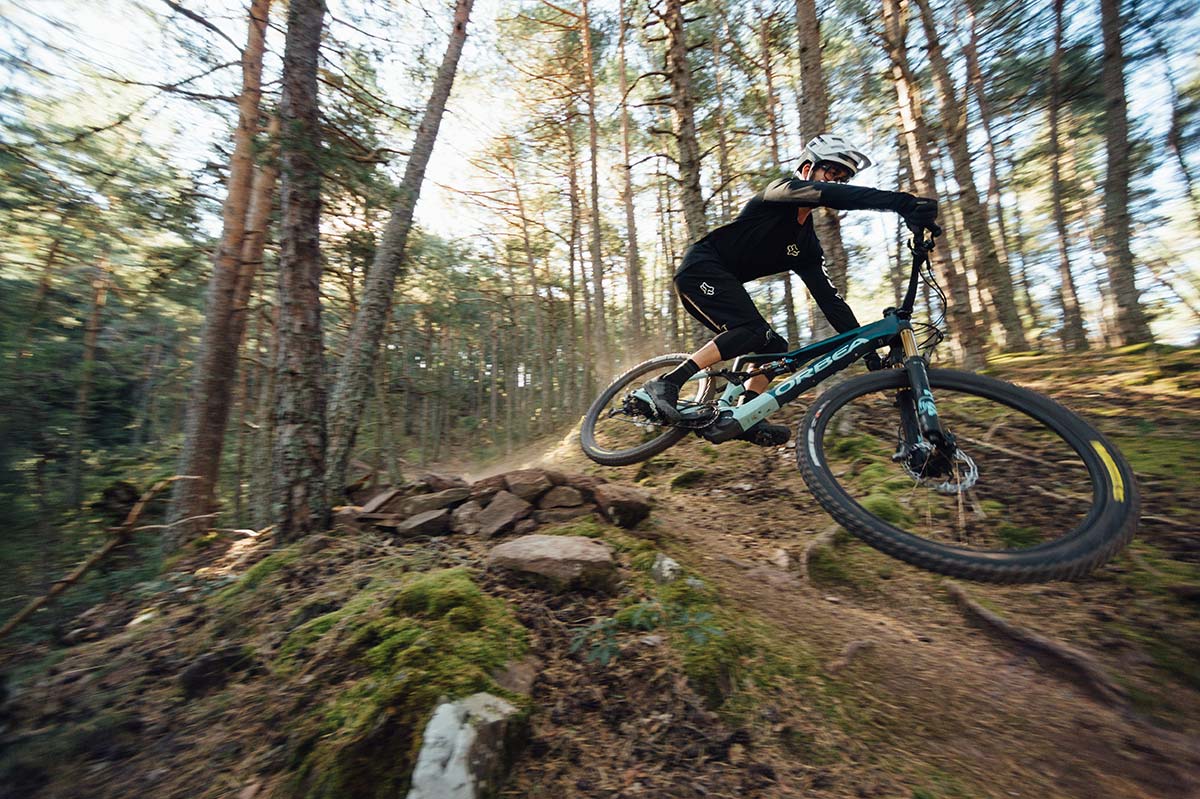In this dynamic daytime photograph set in a dense forest, a cyclist is captured mid-air, having just launched off a rise on a dirt path dotted with rocks and moss. The bike, identified by the Orbea logo, features a forest green frame with a white neck and sports a yellow logo on one of the wheels. The cyclist, likely female, is fully outfitted in black gear including a long-sleeved fitted top, leggings, shoes, gloves, and socks, complemented by a white helmet with black details and black safety glasses. The action shot, focused on the cyclist against a slightly blurred backdrop of slender deciduous and coniferous trees, conveys the high-speed and rugged nature of the trail. The rider is skillfully maneuvering to land the bike after hitting what seems to be a rocky outcropping along this challenging and scenic forest trail.